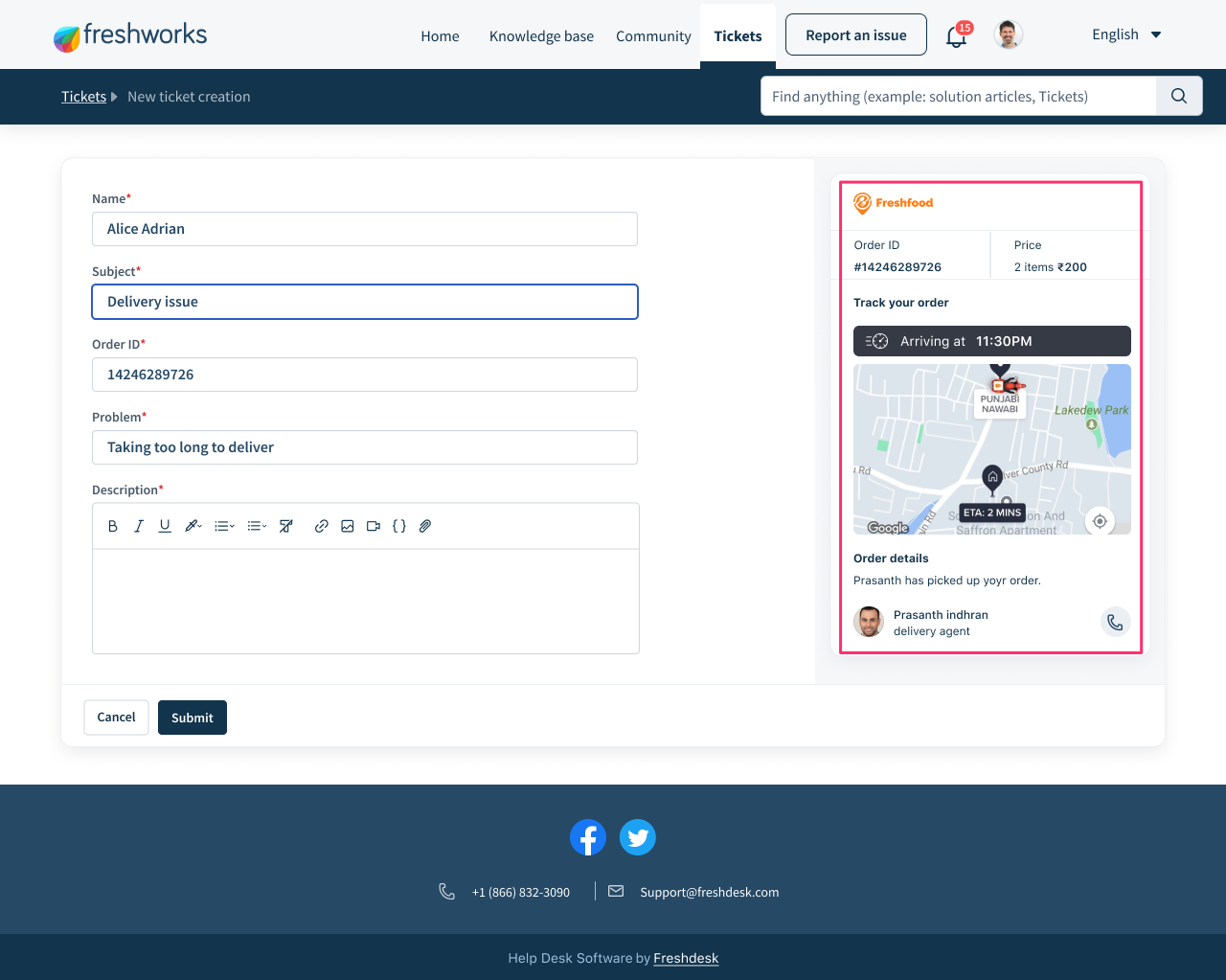Here is a detailed caption based on the provided voice description:

---

This screenshot from Freshworks displays various sections and notifications within the platform. At the top, navigation tabs including Home, Knowledge Base, Community, Tickets, and Report an Issue are visible. A notification icon indicates 50 new alerts. A user profile with a circular picture of a man with short hair appears next to these tabs. The 'Tickets' section is highlighted in a dark green box with an underline and an arrow pointing to it. Below, there's a section titled 'New Ticket Creation' featuring a search box labeled 'Find Anything'. 

This section, set against a white background, includes fields such as 'Name' (Alice Adrian), 'Subject' (Delivery Issue), 'Order ID' with a corresponding number, and 'Problem' described as 'taking too long to deliver'. Alice has just submitted this ticket without filling in the 'Description' field.

To the right, another screenshot captures Alice's order details. The order, placed with 'Fresh Food', includes an order number and the price for two items, totaling over 200. There is an option to 'Track your Order'. A black box above the map displays an ETA of 11:30 PM, noting that the estimated arrival time is two minutes. Further order details mention that the delivery agent, named Password, has picked up the order. A picture and name of the delivery agent are included, along with a phone icon.

---